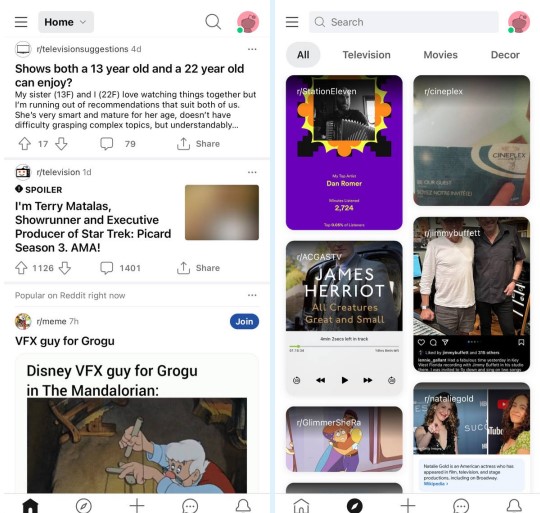The image features two side-by-side Reddit screenshots, highlighting distinct layout differences. The left-hand screenshot is from the Home category and displays subscribed subreddits including Television Suggestions, Television, and Meme. Notably, it showcases three subreddit posts: one indicating both a 13-year-old and 22-year-old can enjoy the content, another under Television from Terry Matalas, the showrunner and executive producer of Star Trek, and a third from the Meme subreddit by a Visual Effects Guy for Grogu. The top right corner of this screenshot shows the user's generic Reddit icon with a green online status indicator.

The right-hand screenshot also seems to be from Reddit but presents subreddits in an icon format. The visible subreddits include Station Eleven, Cineplex, ACGhastie, Jimmy Buffett, Glimmer, and Natalie Gold. This setup contrasts with the left screenshot’s text-based layout, showcasing a variety in Reddit's interface options.